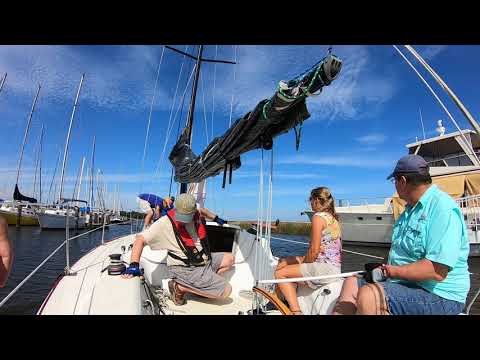The photograph captures a serene moment on a white sailboat, surrounded by a tranquil, partly cloudy blue sky with dispersing wisps of clouds. In the foreground, three individuals are prominently featured. At the center of the image is a man crouched down, his face obscured as he looks downward. He is dressed in a cream-colored hat, a matching cream t-shirt, dark gray pants, and sandals. To his right stands a woman with blonde hair in a shoulder-length ponytail, wearing a fluorescent-colored tank top in yellow and purple hues, coupled with khaki shorts. Further to the right, another man wears a mint-colored collared button-up shirt, blue jean shorts, and a matching blue jean hat, all while facing away from the camera.

The sailboat's primary sail, which is black, is rolled up and secured with a green rope, extending at an angle across the scene from upper right to middle left. The boat's body is white, and a white hand railing is visible on the left side of the frame. In the background, a variety of sailboats, predominantly white, dot the horizon, with a larger yacht featuring a yellow accent to the right. The image is bordered by thick black bands at the top and bottom, giving it a framed appearance. Despite the bustling activity of the sailboats and yachts in the distance, the image exudes a sense of calm and leisurely boat outing on what appears to be a river, with a hint of nature visible in the background.